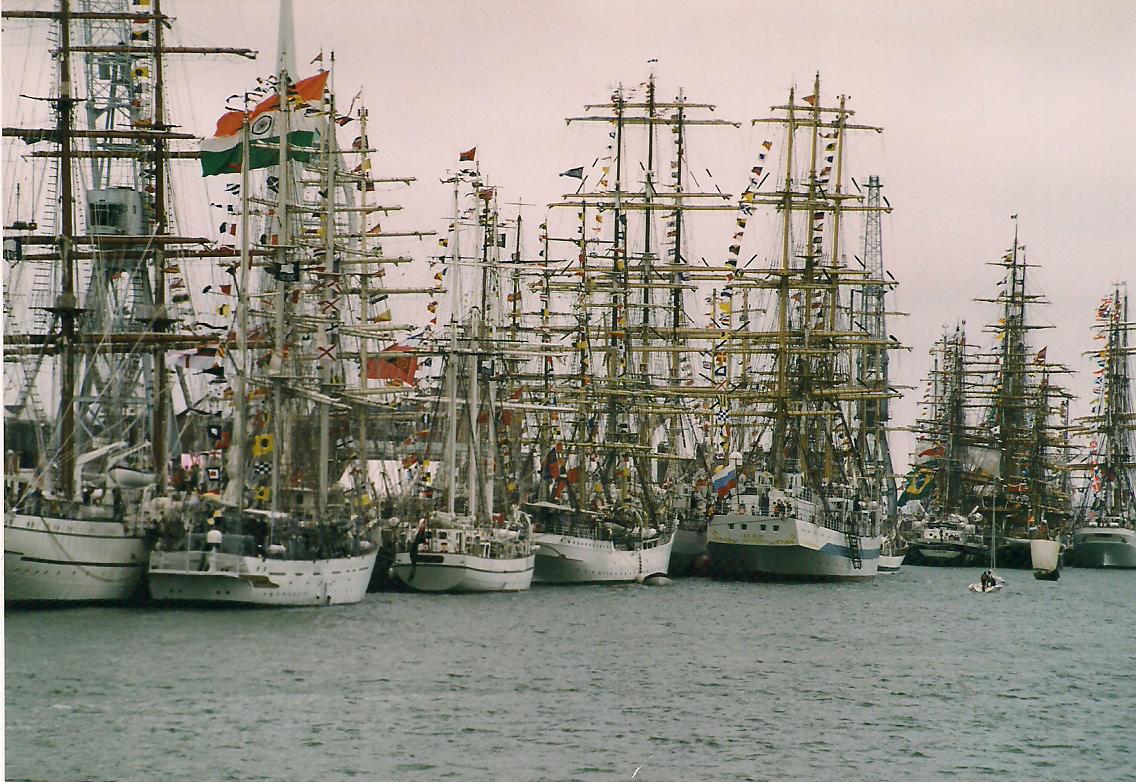The image captures a bustling lagoon or inlet filled with a multitude of sailing ships, predominantly three-masted and two-masted varieties of various sizes. The scene appears to be part of a boating event given the sheer number of ships, which are lined up and stretch far into the distance, creating a dense forest of masts. Among the larger vessels, which sport tall, almost pirate-ship-like designs, there is a smaller white-sailed boat out on the water. The sky overhead is a somber mix of gray and white, contrasting with the light gray and blue hues of the water below. In the background, vaguely visible through the forest of masts, there are hints of buildings or structures, suggesting a nearby settlement. A prominent flag can be seen flying, indicating the location might be in the Middle East, possibly Saudi Arabia or Iraq. This daytime image vividly captures the essence and grand scale of the gathering.